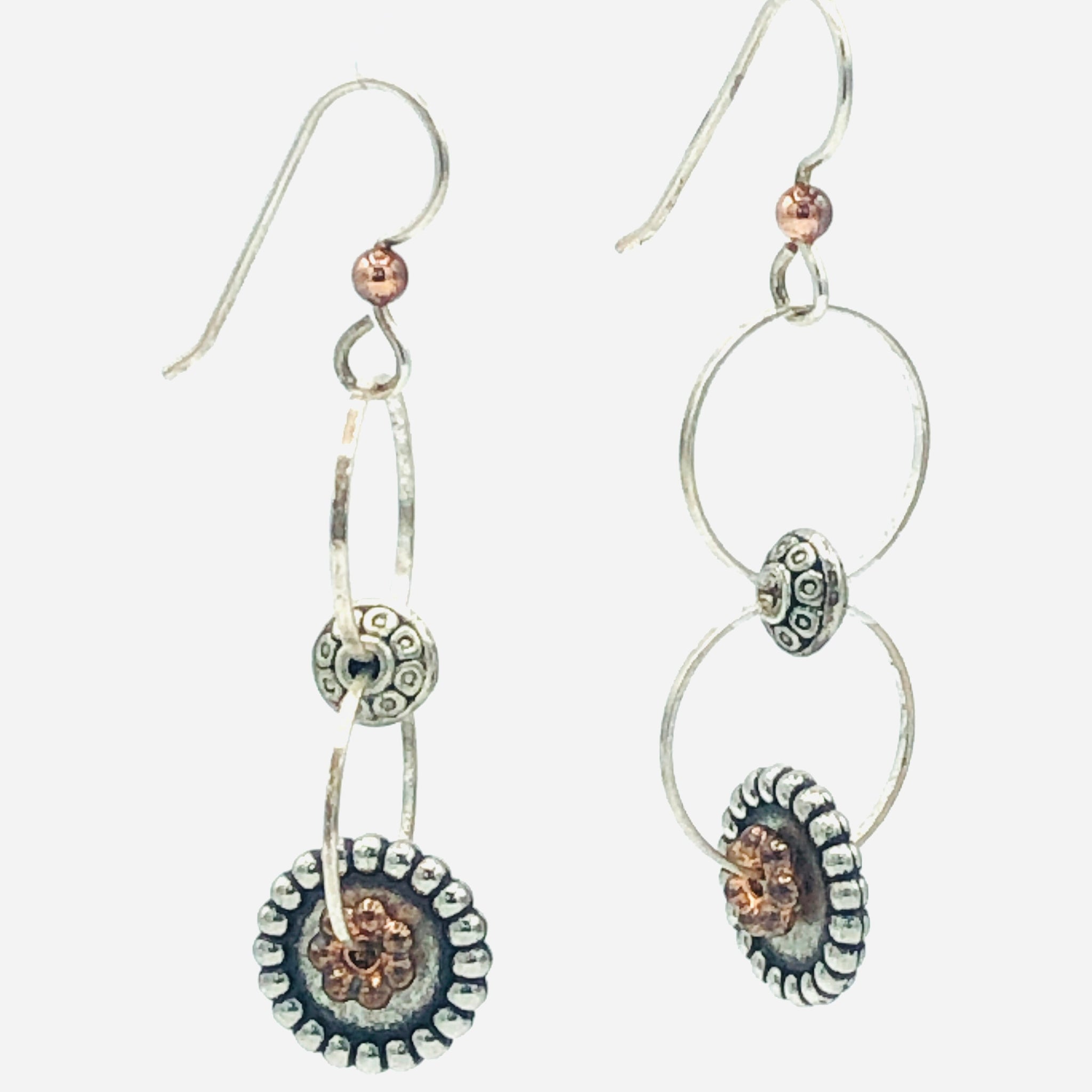This detailed close-up photograph features a handcrafted pair of earrings made primarily from stainless steel and silver, with accents of bronze, copper, and blackened metal. Each earring hangs from a simple, flat, and round silver hook that attaches to the ear. Below the hooks is a small, brass-colored ball and a thin silver loop that connects to a larger, ornate silver hoop. The earrings have a figure-eight design, with two interlinked silver and black hoops. In the center of the arrangement, there is a round, wheel-like piece of silver metal featuring raised details and black accents. Hanging below this is another larger silver hoop, complemented by a second ornate, wheel-like cylinder adorned with raised copper and silver bumps. These long, dangly earrings have intricate craftsmanship yet appear to be lightweight.